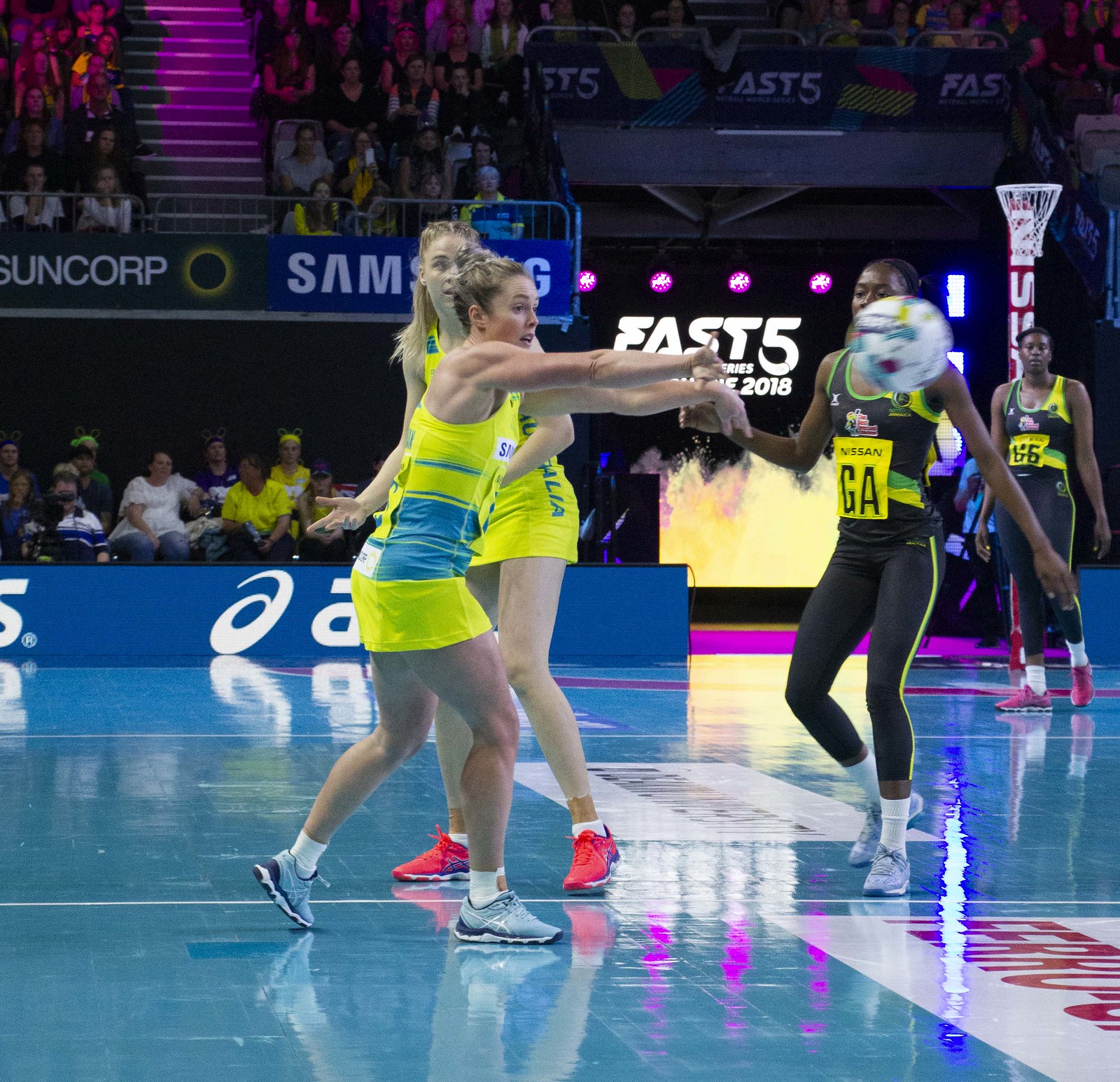The image depicts an indoor athletic event that combines elements reminiscent of both volleyball and basketball. The game is taking place on a large, shiny blue court adorned with ads, including well-known brands such as ASICS, Samsung, and Suncorp, with "Fast Five series" prominently displayed in the background. Multi-level stands brimming with spectators are visible, indicating a popular or significant event. 

In the foreground, a woman in a yellow and blue outfit featuring a tank top and a short skirted bottom is making a dynamic chest pass, her arms extending forward as the ball blurs in fast motion. The ball resembles a volleyball, further adding to the game’s ambiguous nature. To the right, two African-American players clad in black tank tops and stretch slacks intently follow the play. The diverse array of colorful footwear includes pink, blue, and white shoes, adding to the energetic and vibrant atmosphere of the scene. 

Overall, the image captures a spirited sports event featuring two teams in distinctive uniforms, a bustling crowd, and a lively, engaging game that seems to blend the excitement of both basketball and volleyball.